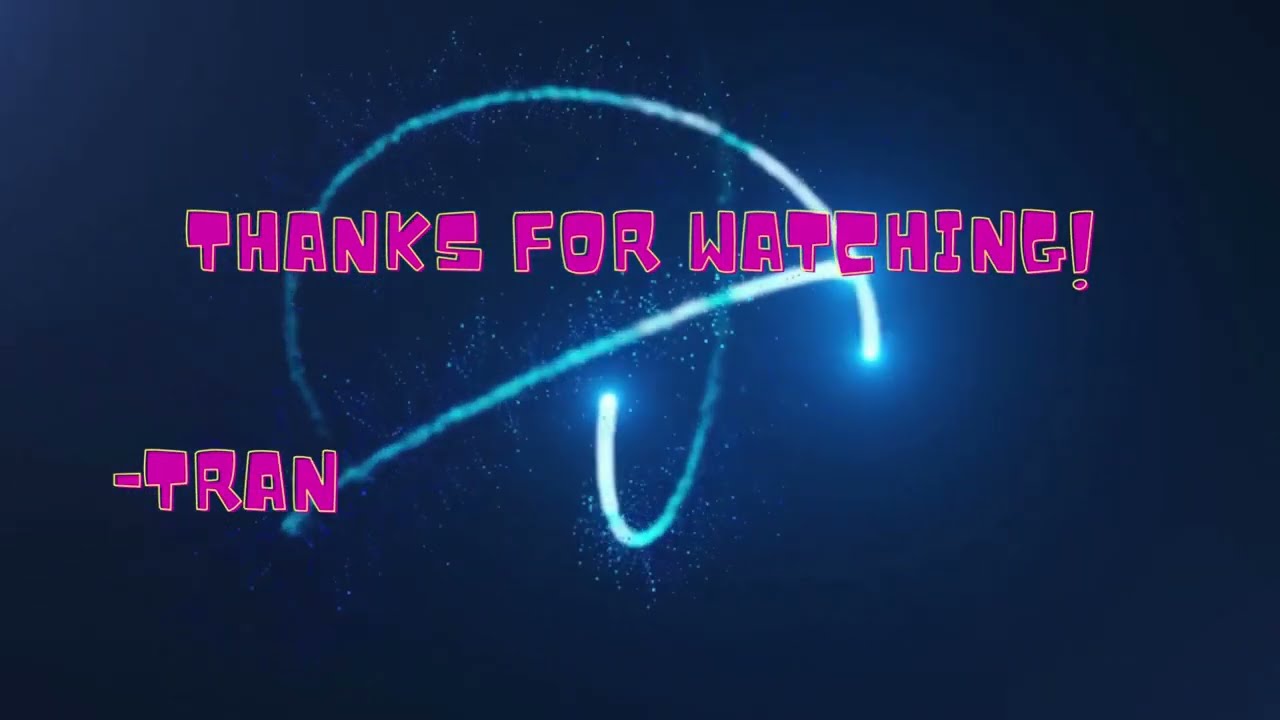The image appears to be a screen grab from a video, possibly YouTube, or a slide from a slideshow. The background is a dark blue, reminiscent of the night sky with teal blue star-like specks scattered throughout. Prominently, there are intricate white, sparkler-like light trails forming arcs: one creating a semi-circle at the top, another swooping from the top to near the bottom, and a third curving from the left up to the right, mimicking the shape of planetary rings in motion. Centered within this celestial backdrop, in bold pink bubble letters with a thin yellow outline, are the words "Thanks for watching," with an exclamation point. Below this text, also in pink, is a simple signature: "- Tran."